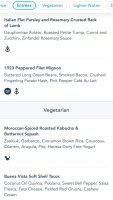The image appears to be a screenshot from a mobile application, given its vertical orientation and mobile-style interface elements. The resolution is very low, making the text difficult to decipher. The background is predominantly white, with a white banner at the top containing pressable buttons outlined in blue and filled with blue text. 

The first button is highlighted, but the text is unreadable. The second button seems to read "Vegetables," and the third possibly includes the word "Lighter," although the exact wording is unclear due to the low image quality.

Below the banner, there is text in black font. One line partially reads "Indian flan" and "rosemary," possibly followed by the word "lamb,” indicated by a small black icon beneath it. Another line mentions "peppered filet." There is a section labeled "Vegetarian," listing items such as "butternut squash" and "coconut oil quinoa," though much of the text is illegible.